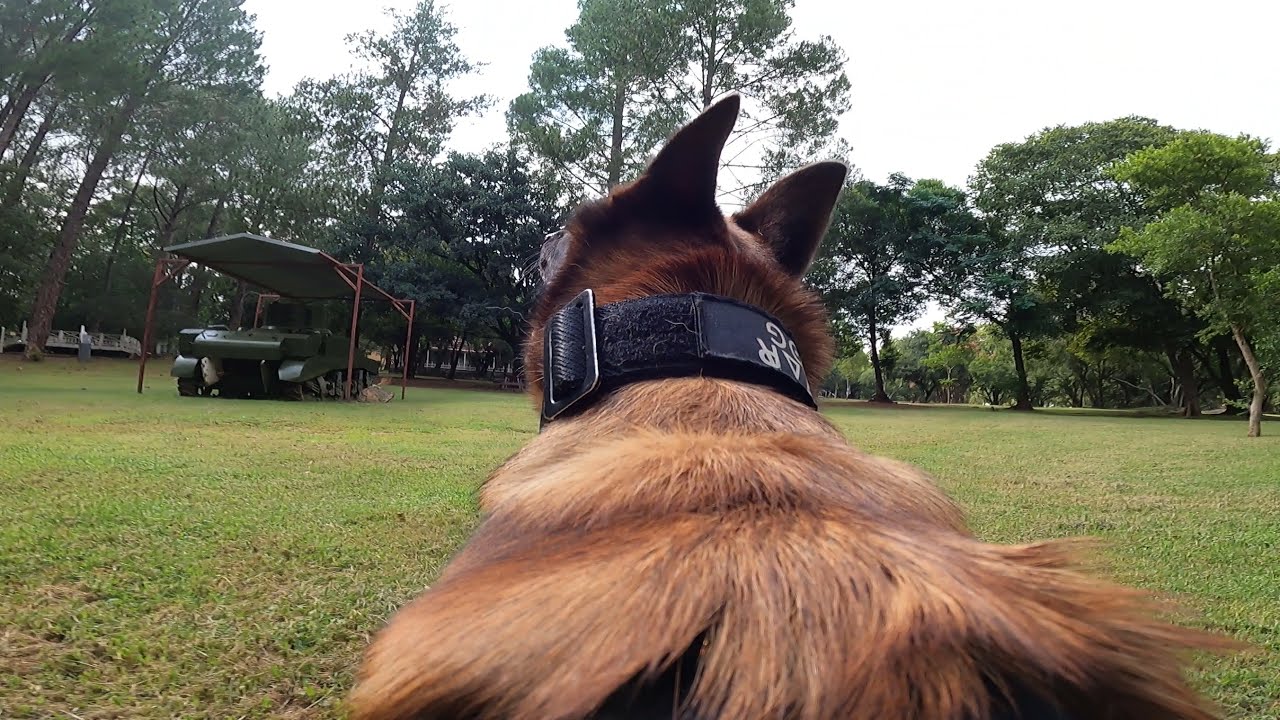This horizontally aligned rectangular picture taken at nearly ground level showcases a lush, well-maintained green grassy area, possibly a park, with a large, open field stretching out behind it. Tall trees with abundant green leaves outline the distant background, reaching up to a grayish-white sky. On the left side of the mid-ground, there's a four-pole carport-like structure with a sheet metal roof, housing what appears to be a small green tank or military vehicle. In the immediate foreground, taking up a significant portion of the lower part of the image, is the backside of a brown and light brown dog, resembling a German Shepherd. The dog is sporting a thick black collar with visible Velcro and a buckle. Only the back of the dog's head, its pointed ears, and the upper part of its body are visible, as it appears to be either standing or sitting, intently facing the tank-covered area to the left. The overall scene is serene, capturing a quiet moment in an open, natural space.